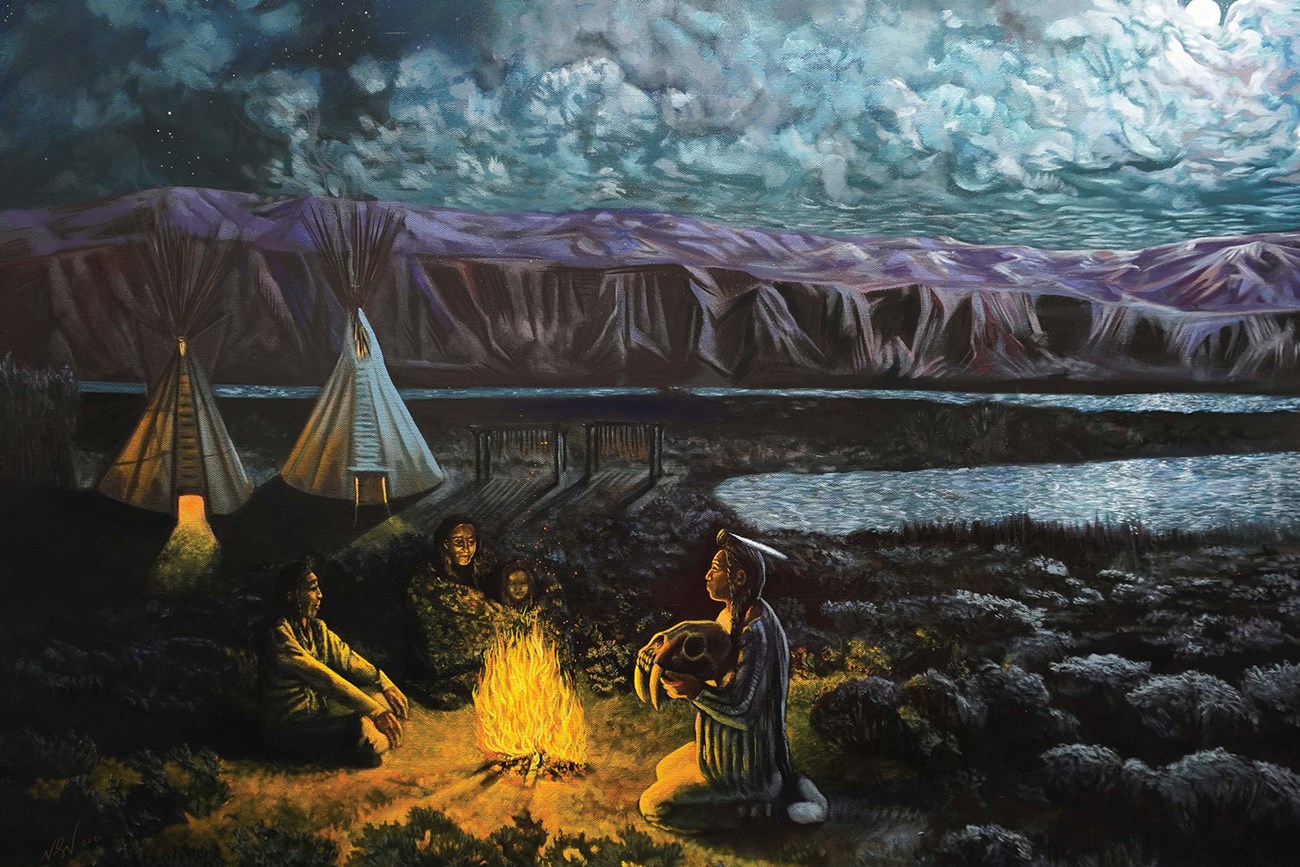In this detailed digital rendering, we observe a nighttime scene depicting four American Indians gathered around a vibrant campfire. The image centers on a woman, child, and two men. One man, positioned to the right of the fire, is kneeling and holding an animal skull with tusks, while the other man sits cross-legged with his arms extended outward. The scene is set against a dramatic backdrop featuring two illuminated teepees. The one on the right appears particularly bright from the inside, suggesting possible occupancy.

The setting includes a dark ground indicative of nighttime, dotted with clusters of blackish-gray bushes on the right side of the image. Behind this, there is a serene lake. Enveloping the entire scene is a sprawling mountainous region, characterized by purple hues and flat-topped peaks that stretch from left to right beneath a rolling expanse of clouds. The sky is richly textured with bluish and whitish clouds, which appear almost glowing, adding a mystical quality to the scene. The darker left side of the sky is adorned with visible stars, contrasting with the middle and right, where the clouds are denser and lighter.